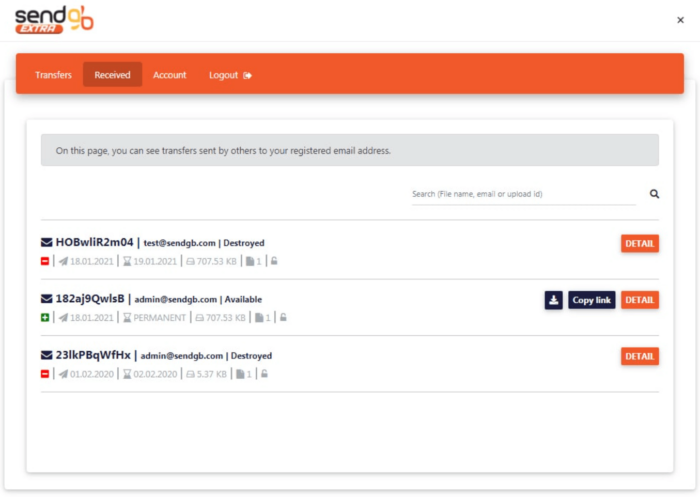The image appears to be a screenshot of a website interface for a service named "Send Extra," as indicated by the orange and yellow logo in the upper-left corner of the screen. Just below the logo, there is an orange navigation bar featuring menu options labeled "Transfers," "Received," "Account," and "Logout." The "Received" option is currently highlighted.

Beneath the navigation bar, a light blue banner provides a brief instructional message: "On this page, you can see transfers sent by others to your registered email address." On the right side of this banner is a search field.

The main content of the page displays a list of three received emails, each represented as a row containing various alphanumeric characters. To the right of each email row is an orange "Detail" button. Notably, the second email row includes two additional buttons next to "Detail": a "Copy Link" button and a button that appears to be for downloading.

The overall design of the interface is straightforward, featuring a white background with black text. The use of orange elements, such as the banner and buttons, adds a contrast that directs attention to interactive components.